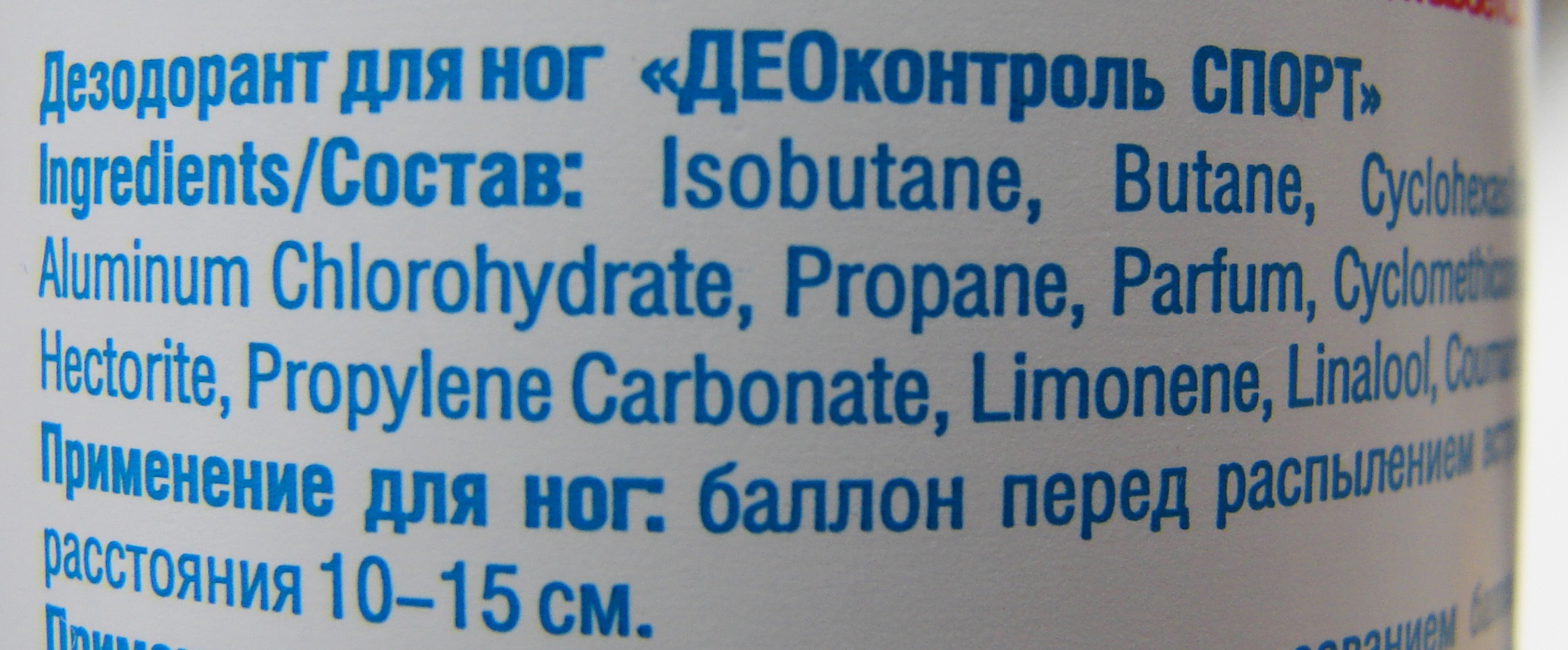The image is a detailed photograph of a white cylindrical bottle, with a white label featuring both English and Russian text that curves around the surface. At the top of the label, blue lettering in a Cyrillic script suggests it is Russian. Below this, in English, the label reads "Ingredients: isobutane, butane, aluminum chlorohydrate, propane, parfum, hectorite, propylene carbonate, limonene, linalool," followed by more Russian writing. Further down the label, it specifies "10-15 cm" along with additional Russian text. The photograph captures this information in a close-up view, making it appear very up close and detailed, emphasizing the curvature of the text on the bottle.